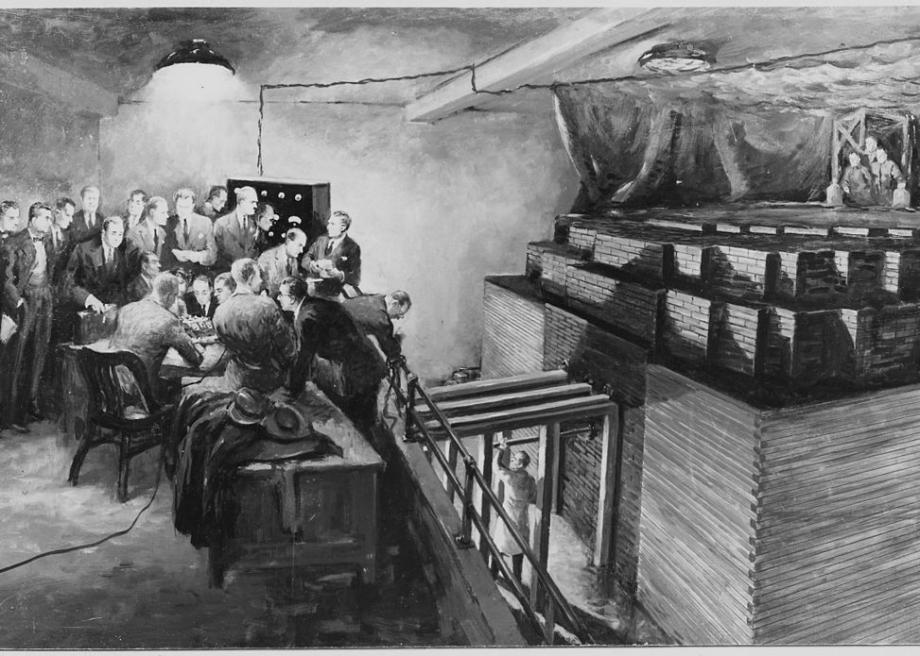This black and white artwork, a combination of pen and ink with watercolor-like shading, depicts a detailed indoor scene that could be a basement, factory, or warehouse. The horizontal, rectangular image is stark and precise in parts, while others have a softer, blurred effect. On the left-hand side, a group of approximately a dozen men in suits and ties are gathered around a table on what appears to be a balcony or higher platform. Some men are standing, while another eight to ten are sitting around the table. Above them, a light hangs from the ceiling, illuminating the scene. Below this higher platform, on the right side, another man can be seen on a lower level near pipes or beams connected to a wall opposite the men. This wall features stacks of bricks and a wooden structure, with additional men visible in the upper right-hand corner, seemingly standing on top of the stacks. The ceiling features large light bulbs and beams running its length, casting numerous shadows throughout the space, adding to the complex and industrial atmosphere.